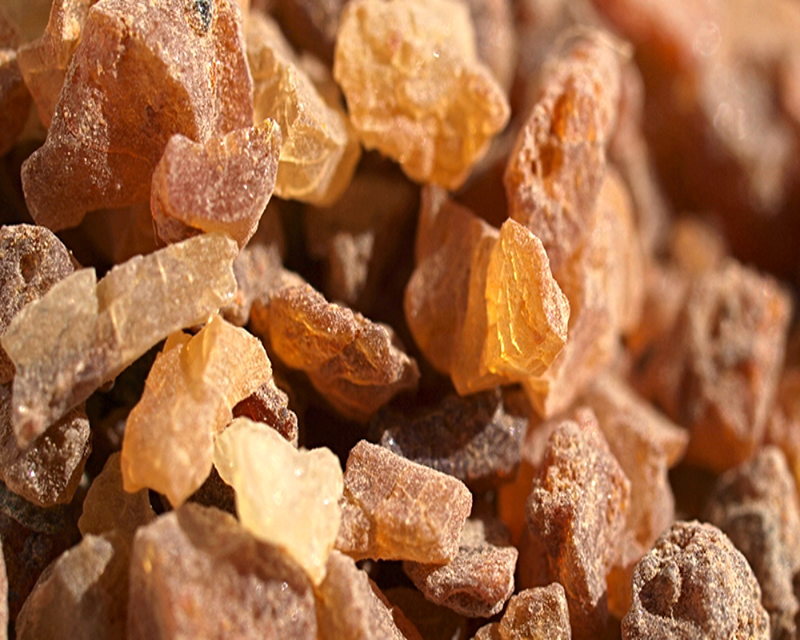The photograph showcases a close-up image of a pile of unfinished stones or crystals, filling the entire frame with no visible background. The foreground features an array of small rocks covered in a dusty, powdery white coating, each varying in shape and size, appearing to be randomly broken. Dominating the upper right corner is a prominent British orange stone, while centrally located near the top is a yellow stone, accompanied by another yellow stone towards the middle. The lower left corner houses a couple of pink stones, with a yellow and pale yellow stone just above them. The bottom right corner is predominantly occupied by pinkish stones, with a couple appearing slightly darker. The image has an amber-hued aesthetic, with colors ranging from golden yellow to dark maroon and darker oranges, evoking a resemblance to natural incense like frankincense. The stones towards the back are blurred, emphasizing the varying texture and unfinished nature of the crystals.